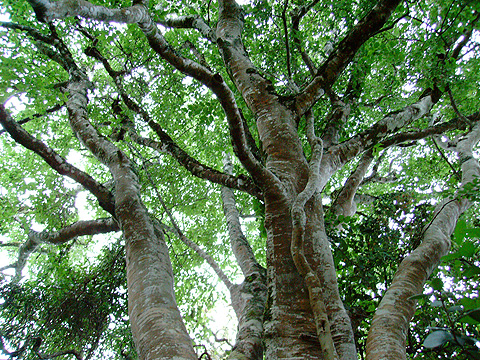The photograph captures an incredibly large, old deciduous tree, viewed from a low angle that gives the perspective of looking up halfway through its impressive structure. The tree exhibits multiple large trunks—four or five—radiating from its base, adorned with many gnarled and intersecting branches. Its bark is a reddish-brown with gray highlights, creating a semi-smooth yet jagged appearance due to its many crooks. The leaves are bright green and abundant, although slightly sparser towards the top, allowing specks of sunlight to filter through. The sunlight peeking through the foliage illuminates the scene with a bright, white light. The sky, partially visible through the leaves, appears light blue. There is a noticeable expanse of white on the trunk, which could be part of the bark or another organism growing on it. The entire tree looks healthy and vibrant, with no visible birds, animals, or man-made objects, highlighting the pure, natural beauty of this potentially climbable tree.